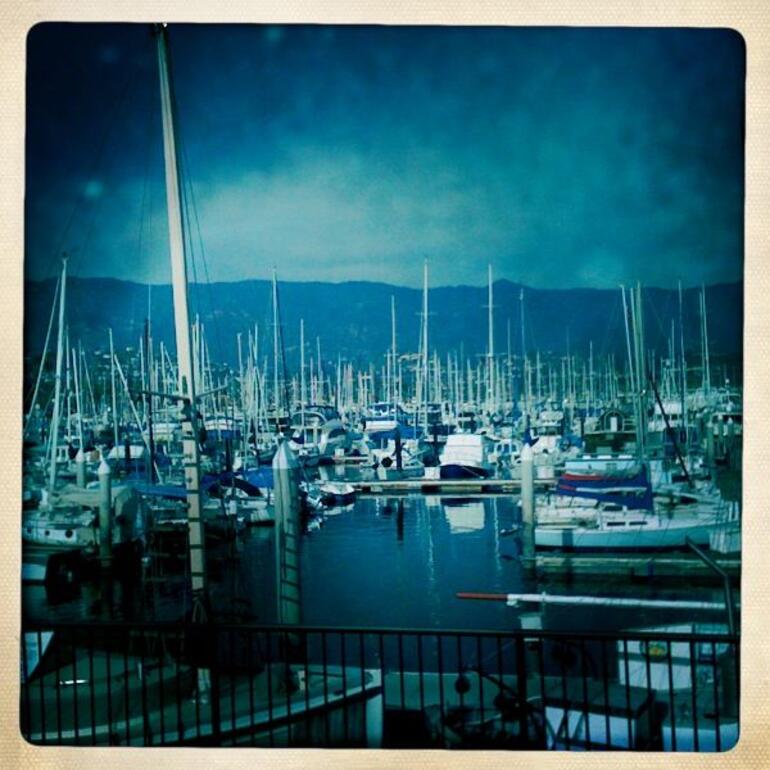The image depicts a dark, foggy or twilight scene in a shipyard or harbor, characterized by a deep blue-black sky gradually transitioning to lighter blue near the horizon. Dominating the background are shadowy mountains tinged with bluish-gray hues. In the forefront, various boats and ships are parked horizontally on the water, with many sporting tall, slender masts that suggest sailboats. These vessels are primarily white, some accented with hints of blue. A black wrought iron fence stretches across the very bottom of the image, partially obscuring potential boxes or containers that might be on a ship just behind it. The overall feel is one of serene complexity, with layered elements of water, boats, mountains, and sky.